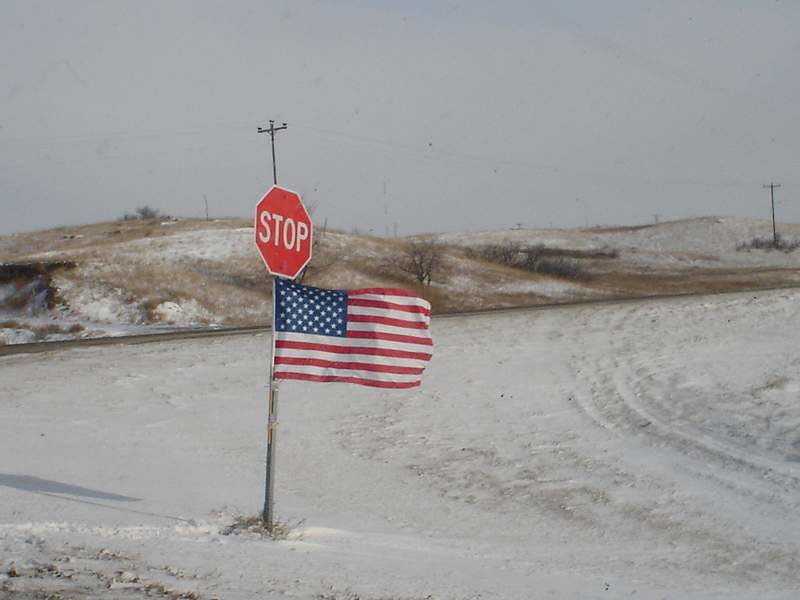In this outdoor daytime photograph, the sky occupies the top half of the image with its light, grayish-white hue, possibly due to haze or light cloud cover. Below the sky, there are small, gently sloping hills dappled with patches of brown dirt and speckled snow. Sparse, leafless bushes are scattered across these hills. Prominent in the middle left section is a large power line pole, with its cables stretching diagonally to another pole situated at the bottom right of the picture. The foreground features a snow-covered road, and at the lower center left, a metal pole stands out, bearing an American flag with its distinctive blue field, white stars, and red and white stripes. Atop the flag, a red, hexagonal stop sign with white lettering commands attention, adding a vibrant pop of color to the otherwise muted winter landscape.